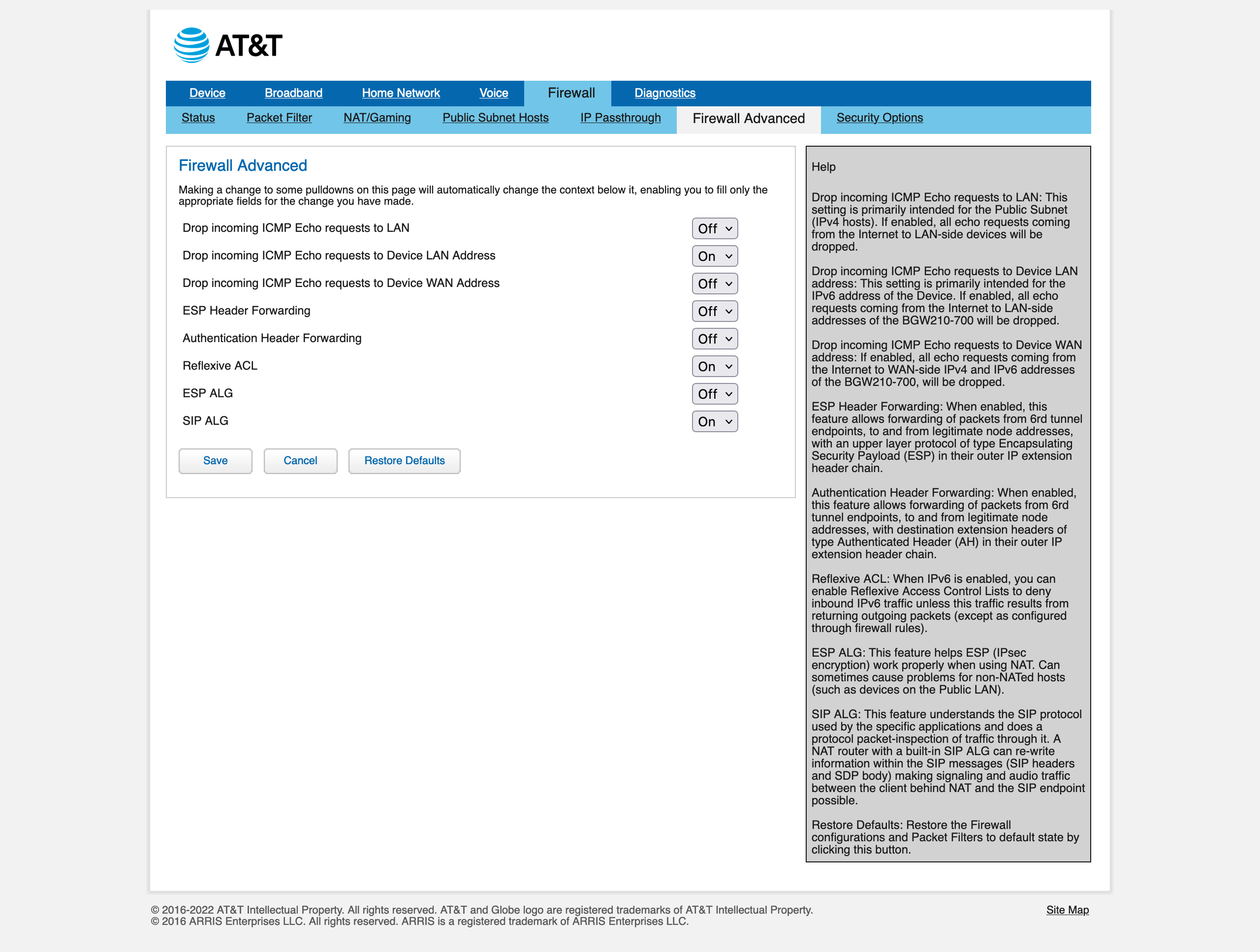**Detailed Caption:**

This image is a screenshot of the Advanced Settings page of the Firewall section for an AT&T modem or router. At the top left corner, the AT&T logo is prominently displayed. The navigation bar features multiple tabs, namely: Device, Broadband, Home Network, Voice, Firewall, and Diagnostics. Within the Firewall tab, there are various sub-tabs that include: Status, Packet Filter, NAT/Gaming, Public Subnet, IP Passthrough, Firewall Advanced, and Security Options. The current selection is the Firewall Advanced sub-tab.

The Firewall Advanced section provides a description stating that changes to the settings can be made using the dropdown menus, with a context-sensitive help section available on the right side for guidance. Visible options include:

- "Drop Incoming ICMP Echo Requests to LAN": Off
- "Drop Echo Requests to Device LAN Address": Off
- "Drop Incoming ICMP Echo Requests to Device WAN": Off
- "ESP Header Forwarding": Off
- "Authentic Header Forwarding": Off
- "Reflective ACL": Off
- "ESP or ALG": On
- "AIP ALG": On

Overall, the image displays a detailed interface allowing users to customize their firewall settings for enhanced network security and performance.